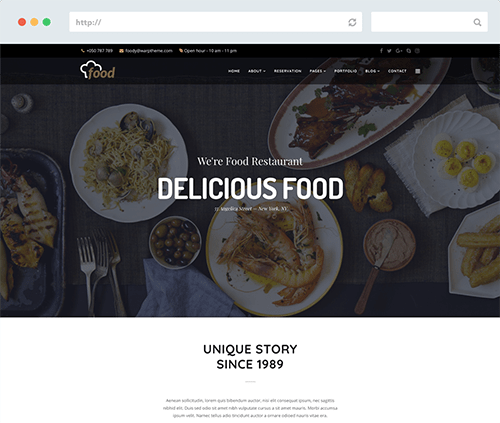This image, captured from a web page, showcases an advertisement for a restaurant named "We're Food." The top section of the page prominently features the website URL, starting with 'HTTP' followed by a 'Colon' and 'Slash slash.' The header of the website displays the word "food" adorned with a whimsical, fluffy chef's hat graphic. Nearby, the page includes the restaurant's phone number and other contact details. Navigation options are visible, such as an 'About' link and several clickable tabs with drop-down menus. The typography varies in size and prominence; "we're food restaurant" appears in a moderate font size, while "delicious food" is emphasized in bold, all-capital white letters, making it the most eye-catching text on the page. Additionally, the background subtly highlights the text "unique story since 1989," and there is very small print located at the bottom of the image.